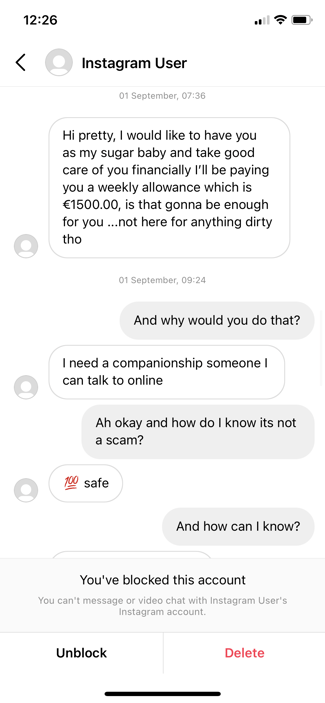This image is a screenshot of an Instagram direct messaging conversation. At the top, there is a backward arrow icon, and a small, faceless purple avatar representing a generic Instagram user is visible. The conversation is initiated by the user named "Instagram User" who sent a message on September 1st at 7:36 PM, expressing a desire to establish a financially supportive relationship. The message reads, "Hi pretty, I'd like to have you as my sugar baby and take good care of you financially. I'll be paying you a weekly allowance, which is $1500. Is that going to be enough for you? Not here for anything dirty though."

In response, the recipient inquires, "And why would you do that?" The sender answers, "I need companionship, someone I can talk to online." The recipient then questions, "Okay, and how do I know it's not a scam?" The sender attempts to reassure the recipient by stating, "100% safe."

The conversation abruptly ends with a notification bar appearing across the screen, indicating that the account has been blocked by the recipient.